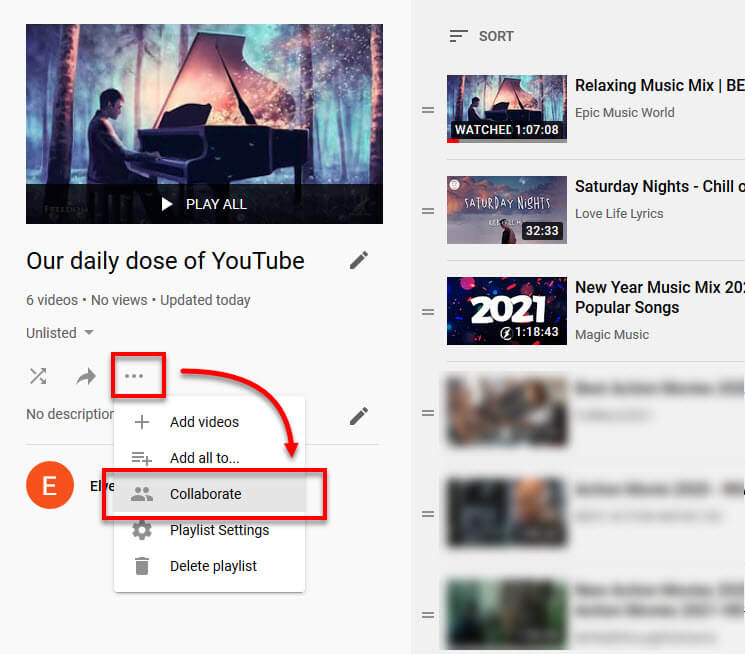Here's a detailed and cleaned-up caption for the image:

---

A screenshot from YouTube features an illustrated image of a man seated between trees in a forest, playing a piano that emits a gentle glow. In the top left corner, it indicates "Our Daily Dose of YouTube" with six videos, zero views, and updated today, marked as unlisted. Three horizontal dots are displayed beside this information within a red square and an arrow pointing to the "Collaborate" option in the dropdown menu. Above "Collaborate", the menu includes options like "Add Videos" and "Add All To", while below it, "Playlist Settings" and "Delete Playlist" are listed. An orange circle with a capital E is positioned to the left of the dropdown menu. On the right, a list of videos is visible with sorting options at the top. The playlist includes titles like "Relaxing Music Mix", "Saturday Night Chill", "New Year Music Mix", and "Popular Songs".

---